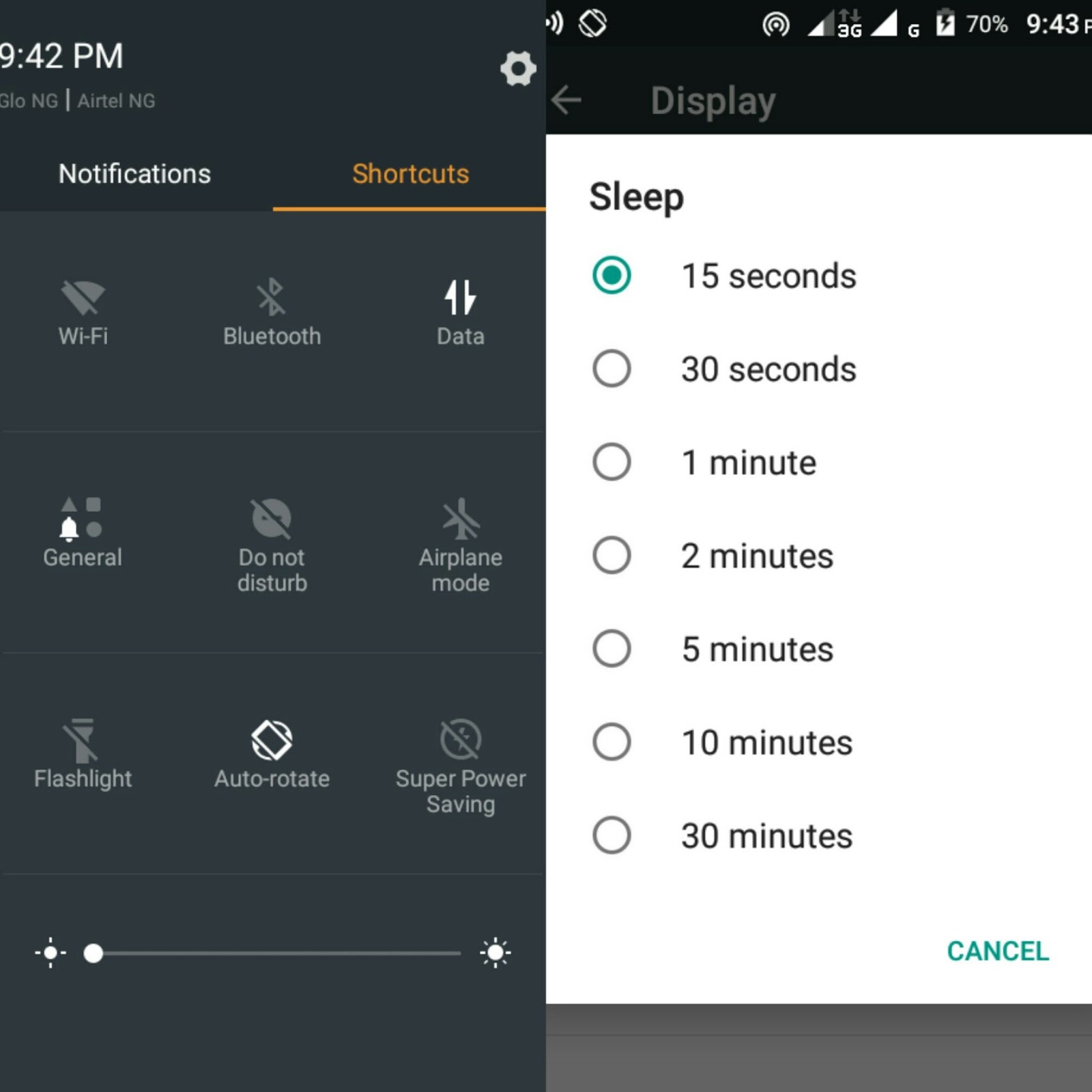The image depicts a settings interface on a smartphone, likely an older model, as indicated by the 3G icon at the top. The screenshot shows two distinct sections with contrasting backgrounds and functionalities. 

On the left side, against a dark background, several settings options are listed: Notifications, Shortcuts, Wi-Fi, Bluetooth, Data, General, Do Not Disturb, Airplane Mode, Flashlight, Auto-Rotate, and Super Power Saving. 

On the right side, a menu related to screen sleep settings is displayed with a white background and black text, showing options for sleep timing intervals: 15 seconds, 30 seconds, 1 minute, 2 minutes, 5 minutes, 10 minutes, and 30 minutes.

Notably, the screenshot also reveals a discrepancy in the device’s clock display, with the top bar showing '70% 9:43 PM' while the left section displays '9:42 PM.' The service providers mentioned are 'Glow NG' and 'Airtel NG.'

This clear division between the dark and light backgrounds, accompanied by the difference in time stamps, suggests that the image might be a compilation of screenshots taken at different moments.